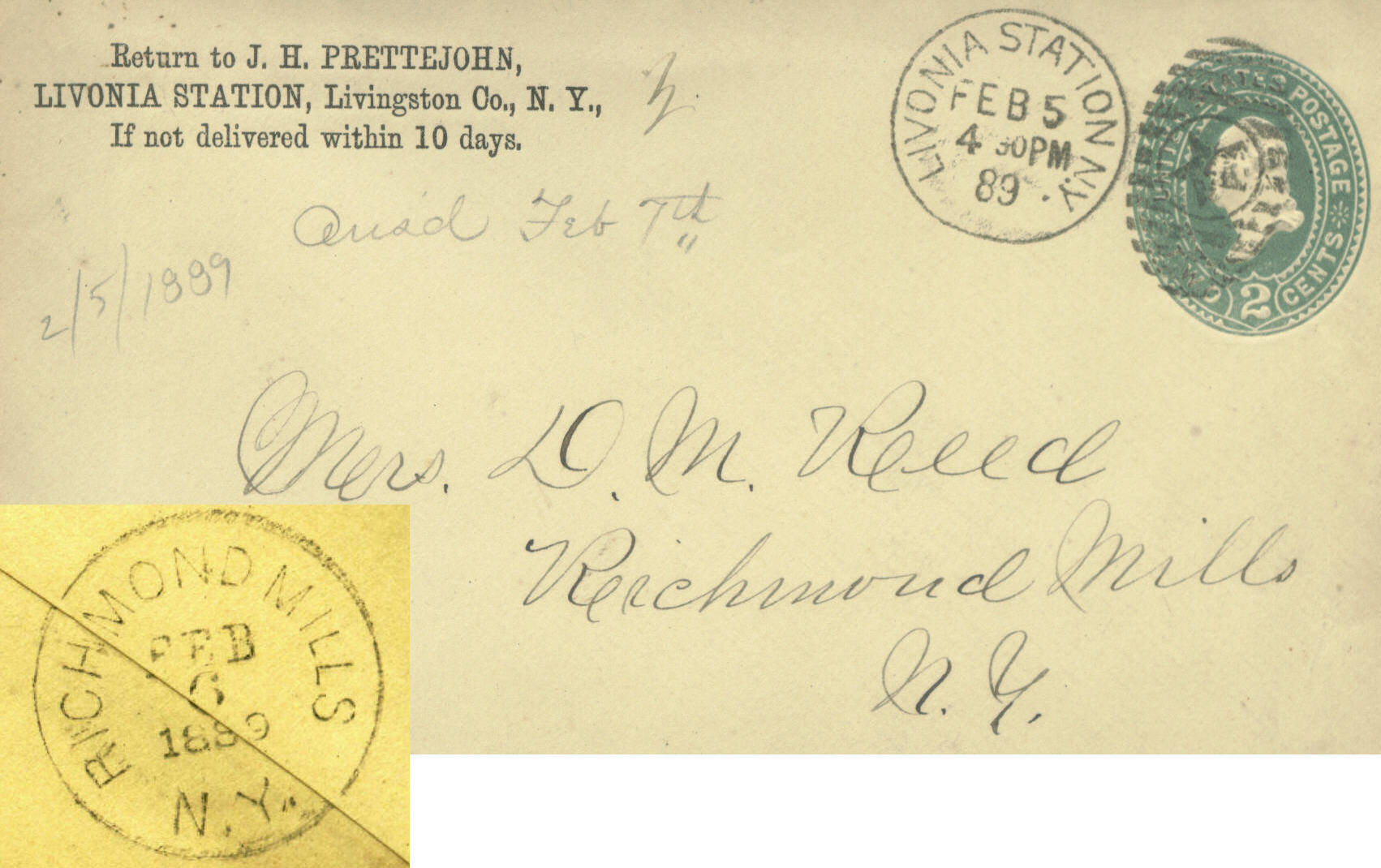The image depicts an old letter against a beige backdrop. In the upper left corner, there's a return address that reads, "Return to J.H. Prettejohn, Livonia Station, Livingston County, New York, if not delivered within 10 days." On the top right side, several postage stamps are visible. One of the stamps is green with a white profile of a human face, marked "two cents." Another stamp is a round circle that reads, "Livonia Station, February 5, 4:30 p.m., 89." Handwritten in elegant cursive on the letter, it states, "2-5-1889, Mrs. D.M. Reed, Richmond Mills, New York." Additionally, in the lower left corner, there's a yellow square seal that says, "Richmond Mills, February 1889, New York." The photo offers a detailed close-up scan, capturing the vintage essence and intricate details of this historical correspondence.